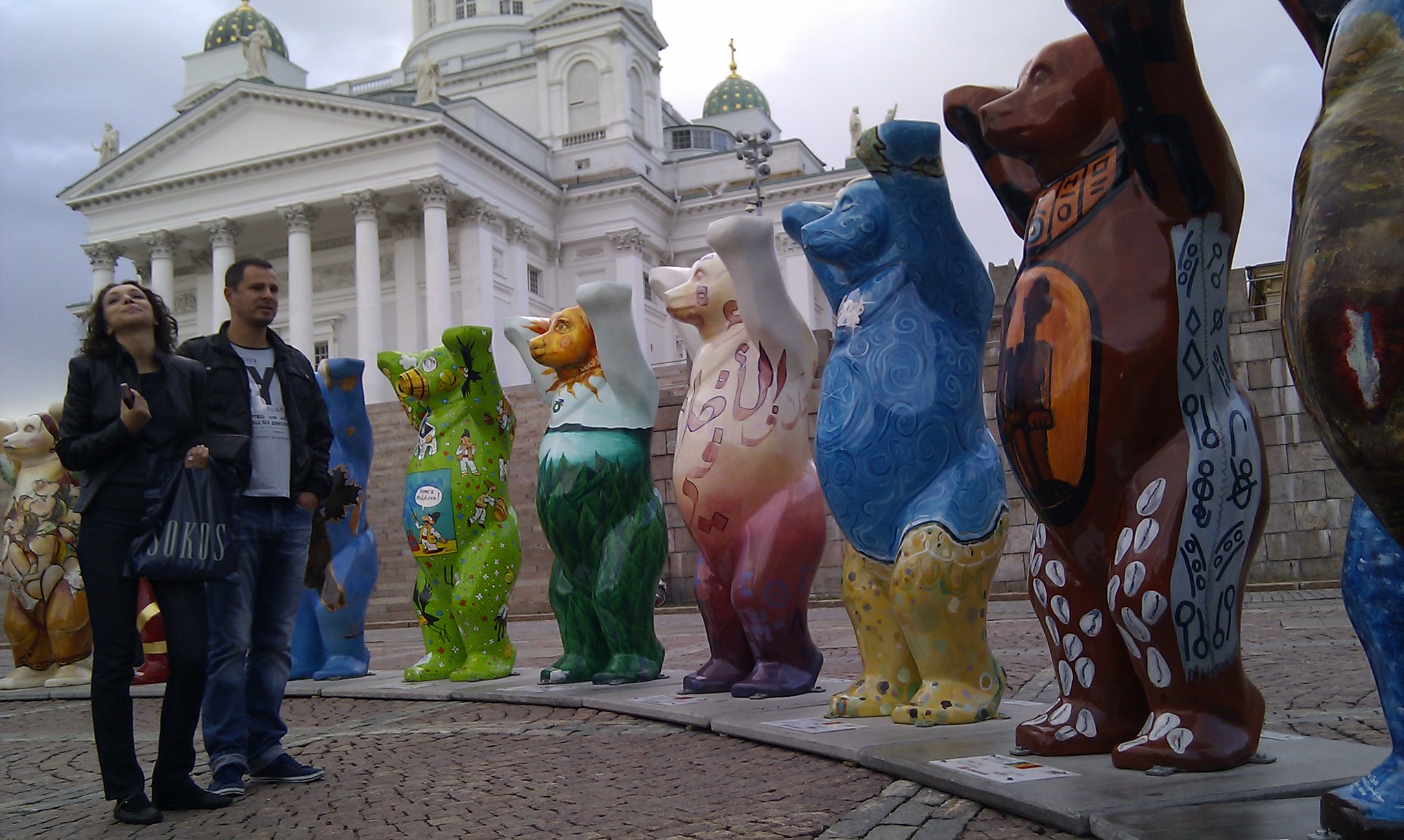The photograph captures an outdoor scene featuring a grand, classical Greek-style building with white columns and green-domed roofs that could be a church or government structure. The sky above is filled with white and gray clouds. In the foreground, there's a cobblestone street and a sidewalk where a man and a woman stand. The man, wearing blue jeans, blue sneakers, a white T-shirt with writing, and a jean jacket, stands next to the woman, who is dressed in black pants, black shoes, and a black blazer, holding a bag that says 'SOKOS'. They are surrounded by a semi-circle of life-size bear statues, each uniquely decorated with various bright, colorful patterns. These bears, with arms raised, are painted in shades of green, pink, blue, brown, and more, contributing to a vibrant, eclectic display likely part of a massive art project. The statues create a stark contrast against the majestic white building and the drably dressed couple, adding intrigue to the historical setting.